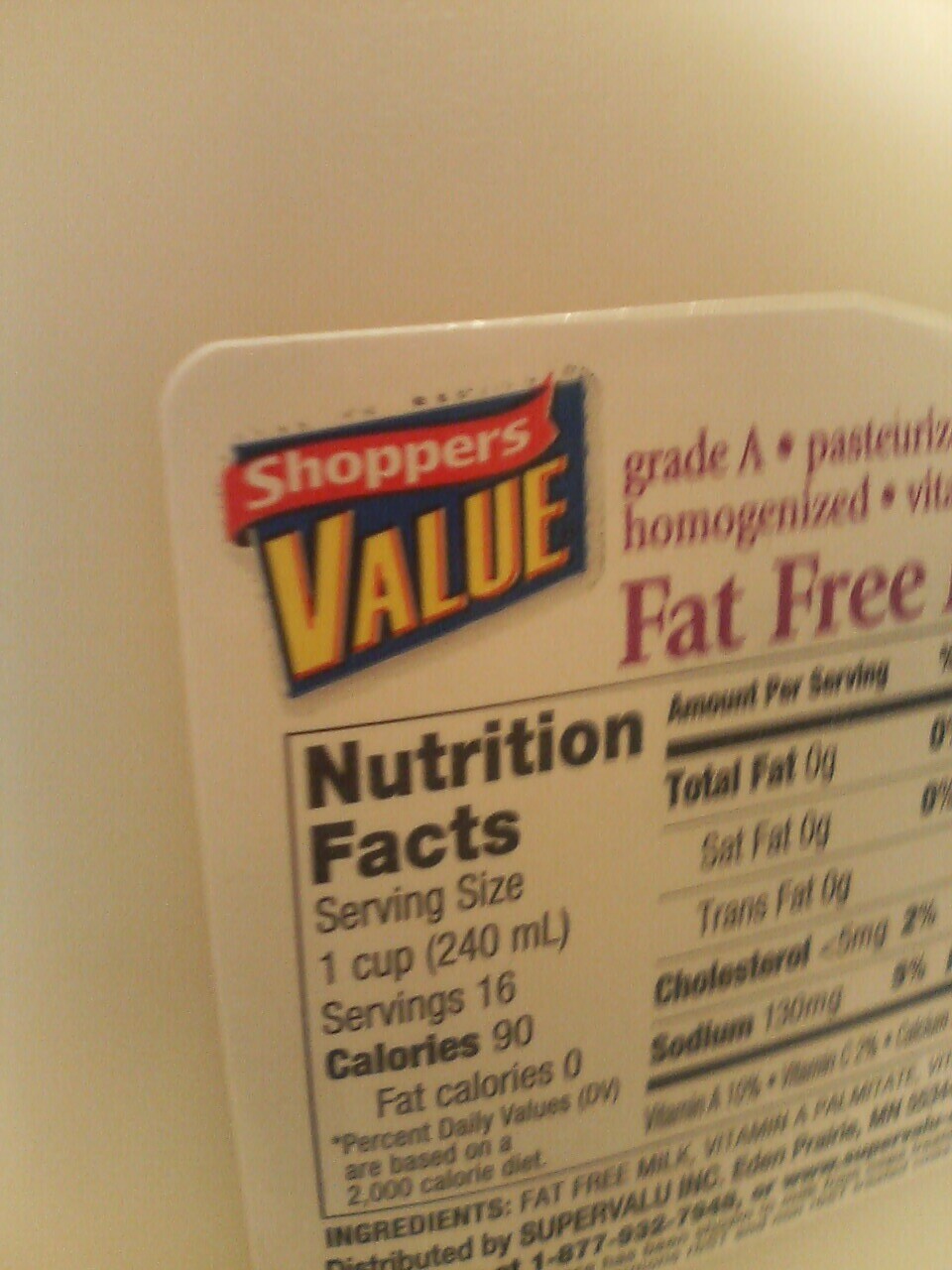This photograph features a packaged food product prominently labeled "Shoppers Value." At the top of the image, a red ribbon with white text displays the word "Shoppers," followed by the word "Value" in gold font below it. 

Clearly outlined in red font, the product is described as "Grade A Pasteurized, Homogenized, Fat-Free." Adjacent to this description, a nutrient label provides detailed information. The label, primarily white with black text, states: 
- Serving size: 1 cup (240 ml)
- Total servings: 16
- Calories per serving: 90
- Calories from fat: 0
- Total fat: 0 grams
- Saturated fat: 0 grams
- Trans fat: None
- Cholesterol: 2%
- Sodium: 130 milligrams

Further down, an ingredient list begins with "fat-free milk and vitamin A," though the remainder of the list is partially cut off in the image. 

At the bottom of the label, it is noted that the product is distributed by Super Value Inc., followed by a contact phone number. This carefully packaged item is presented in a manner that highlights its nutritional benefits and adherence to rigorous quality standards.